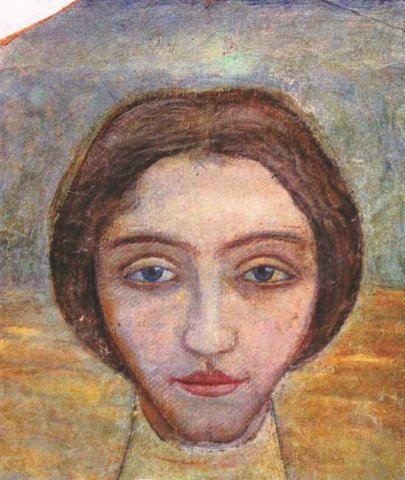The image is a detailed, colored sketch of a woman’s head and neck. Her hair, brown and wrapped around her ears, flows down into a low bun that covers her ears from view. She has large, round, and slightly mysterious grayish-blue eyes, a nose with a slight ridge and a rectangular tip, and closed lips that are light pink in color with the top lip being wider than the bottom. Her neck is long and adorned with a yellow turtleneck. The background transitions from an orangey-yellow below the ear section to a light green and gray above it, with a hint of golden brown at the bottom and a bluish-gray mix up top. The top left corner reveals a bit of white canvas of the rough-textured backdrop.